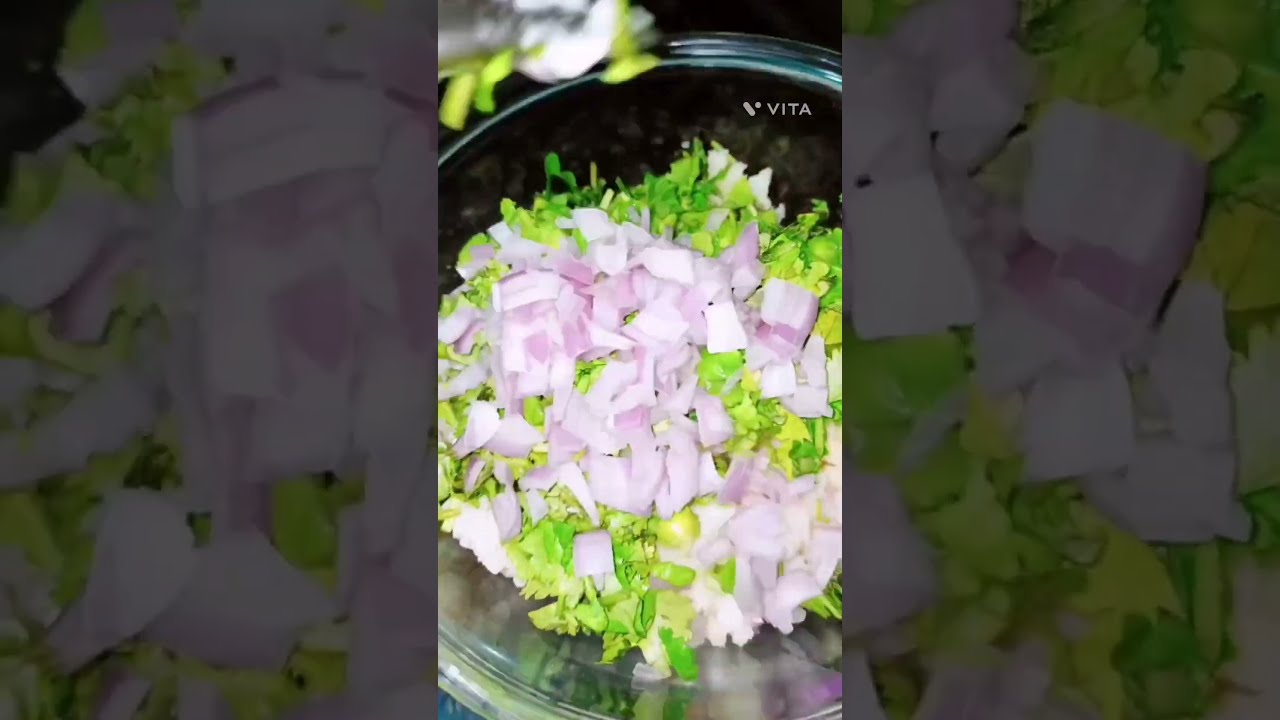This is a cell phone image of a partially visible clear container holding chopped vegetables, hinting at a salad in preparation. The main focus is on the upper section of the container, where chopped green lettuce and what appears to be pink and white onion pieces are prominently displayed. A grayish watermark reading "VITA" is located at the top right of the image. The photo shows no hands or people, suggesting a solitary setup, potentially for a cooking show. The background features shadowed, darker images flanking either side, slightly larger, emphasizing the sharpness of the central image. Overall, this picture captures an intimate, zoomed-in view of fresh, vibrant vegetables ready to be mixed.